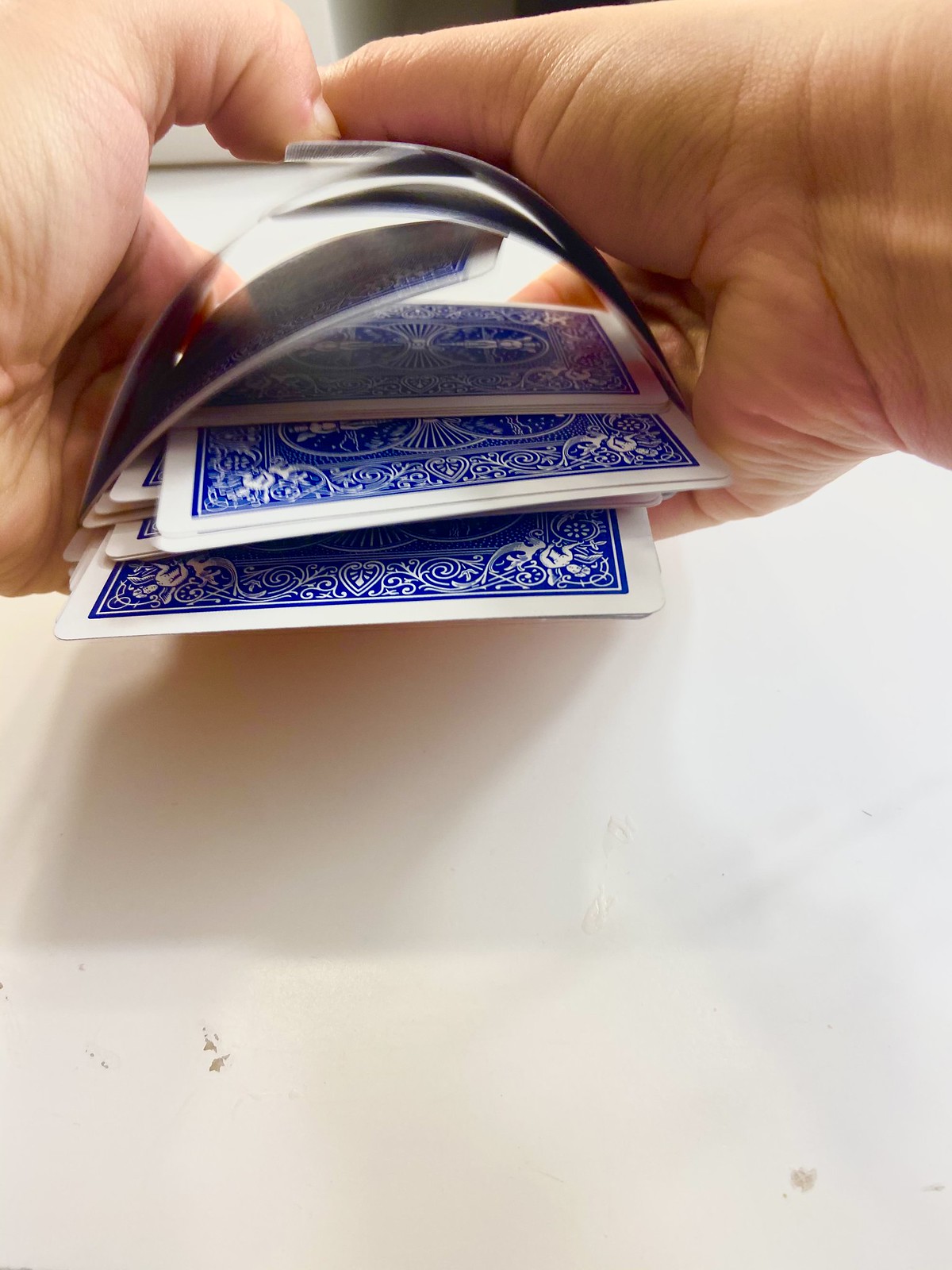The image captures the action of someone skillfully shuffling a deck of playing cards. From a first-person perspective, two hands are visible emerging from the upper left and right corners, converging in the center where a small stack of cards is held. The cards themselves feature an intricate blue and white design adorned with swirls, hearts, spirals, and what appear to be angelic figures. This scene unfolds over a white desk or tabletop, which shows signs of wear and tear, with scuff marks revealing the wood beneath the paint. The lighting, seemingly overhead, casts distinct shadows of the hands and cards onto the table's surface, adding depth to the image. The cards are captured mid-shuffle, some of them arched in mid-air, showcasing the dynamic movement as they fall and rearrange into the deck.